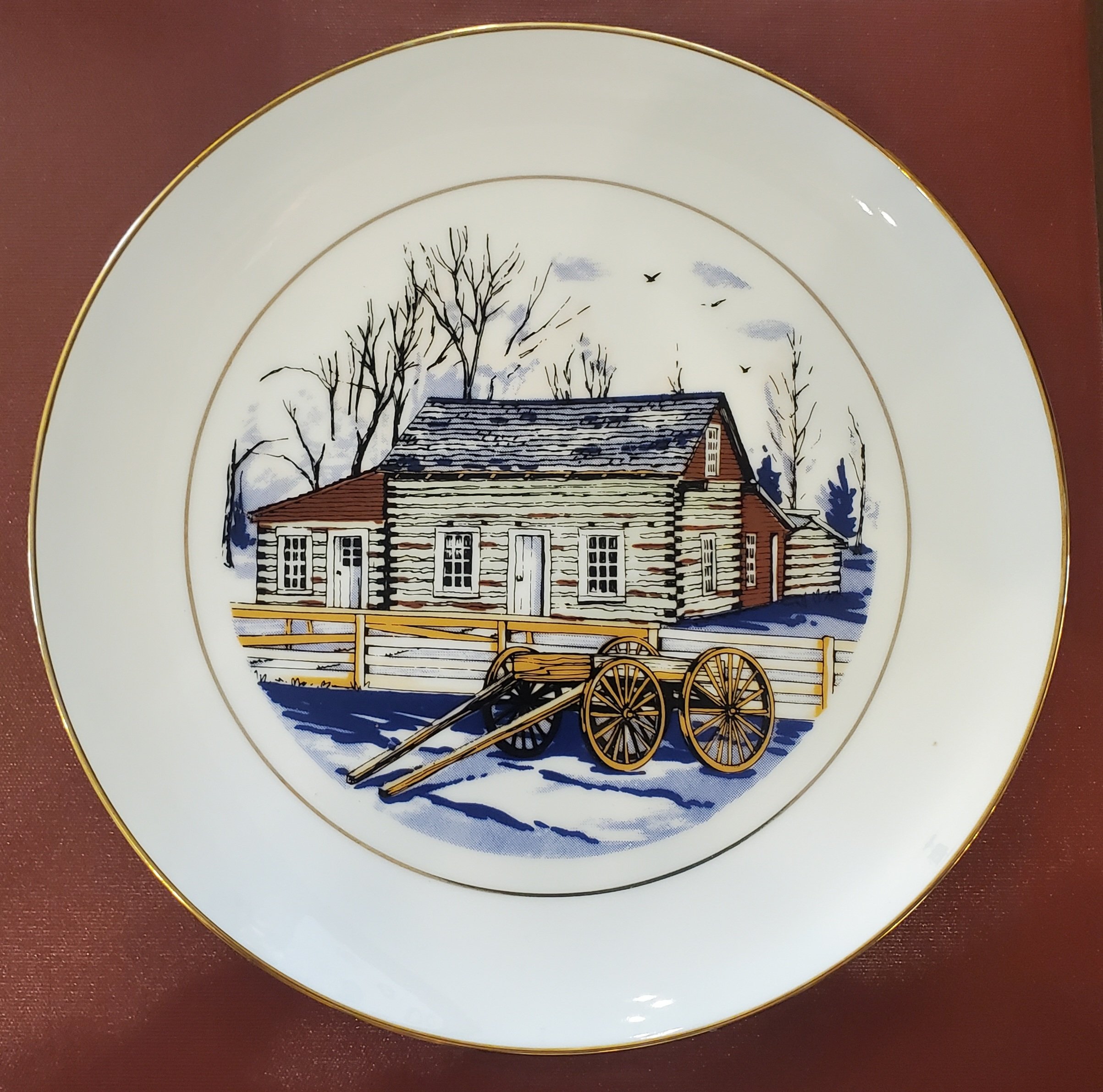This detailed china plate is an exquisite decorative piece. Its glossy white surface is elegantly framed by a thin gold rim along the outer edge and another concentric gold ring toward the center. At the heart of the plate is a detailed illustration of a log cabin surrounded by a picturesque winter scene. The log cabin features a cream-colored facade with contrasting darker wood parts and a black roof, accented with hints of reddish shades. The cabin has four or five windows and two doors, suggesting a quaint and rustic charm. In the foreground, there is a slightly dilapidated wooden fence and an old wooden carriage or wagon positioned before it. Surrounding the cabin are bare trees, a few scattered birds, and fluffy clouds in the sky, all set against a bluish-gray ground covered with patches of snow.